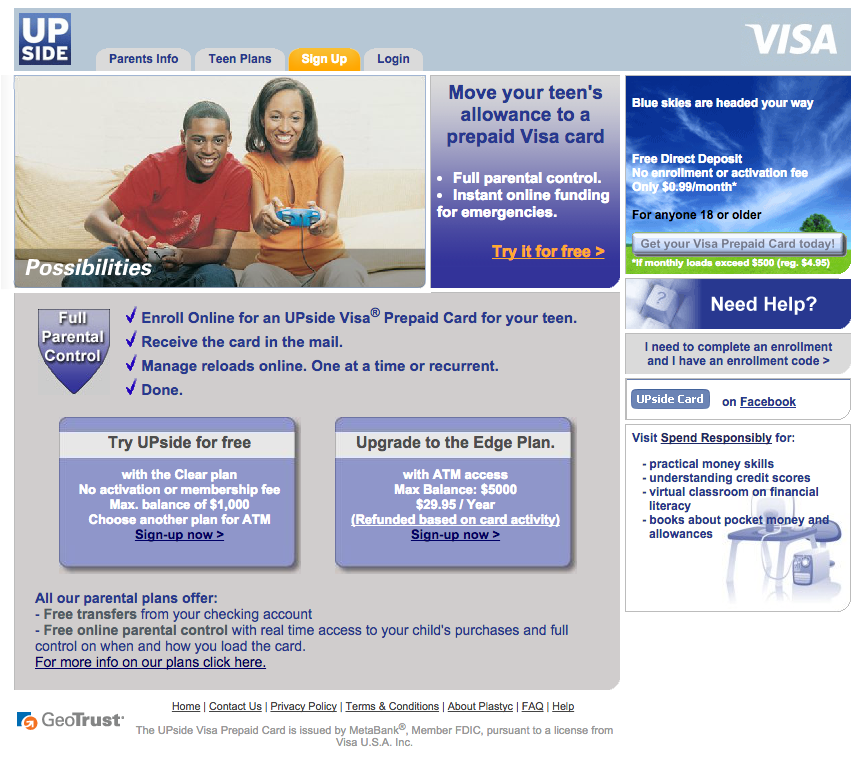This web page features a comprehensive section with links for easy navigation including 'Parent Info,' 'Team Plans,' 'Sign Up,' 'Log In,' and 'Possibilities' situated in the top left corner. The main visual highlights a young boy engaging in a game with his mother. Near the mother, a text bubble suggests action: "Move your team's allowance to a prepaid Visa card." The caption emphasizes full parental control and lists benefits such as instant online funding for emergencies, free direct deposits, and no enrollment or activation fees. A call-to-action prominently invites users to "Try it for free," also mentioning an affordable monthly fee of $0.99 for users 18 years or older. Additional incentives are specified for users with monthly loads exceeding $500. For assistance, there's a mention of completing an enrollment using an enrollment code, and the invitation to follow 'Upside Card' on Facebook. The footer encourages responsible spending with practical money management skills.